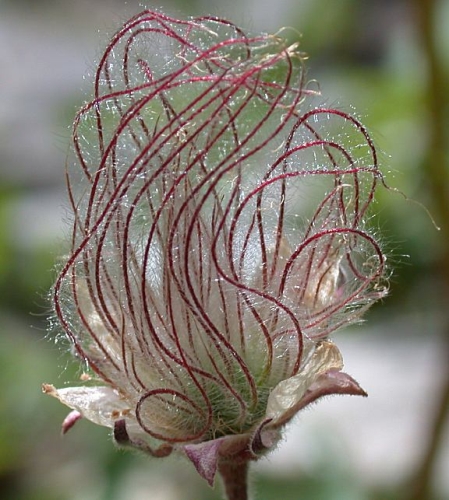The image captures an outdoor scene with a vivid flowering plant as the focal point. The blossom, resembling a flower with a mix of purple and magenta strings or tentacles, extends upward in a curling, snake-like fashion. These tendrils are maroon-colored and covered in fine, glistening hairs, reminiscent of fiberglass filaments catching the sunlight. The base of the plant features a fuzzy stem with small mauve and white petals. In the blurred background, green leaves from other plants create a lush, out-of-focus backdrop, adding depth to the scene and emphasizing the intricate details of the flower in the foreground. The entire composition is captured outdoors, bathed in natural light, enhancing the vibrant colors and textures of the plant.